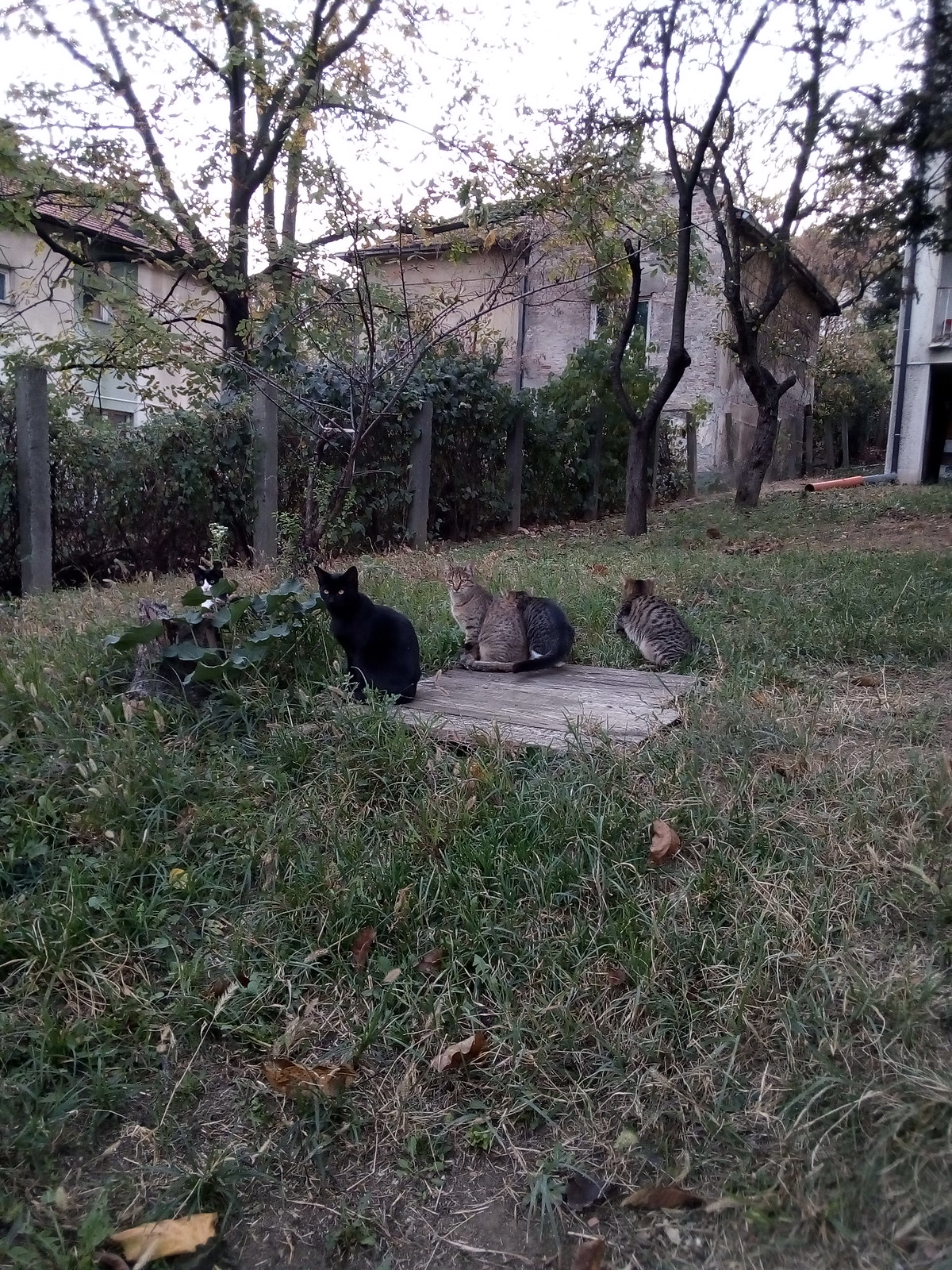This is a color photograph taken outdoors, capturing a muted, almost wintry scene in what appears to be a backyard in a residential area. At the center of the image, five cats sit clustered together on a square patch of grey wooden planks positioned in the middle of brownish, slightly overgrown grass. Among the cats, there is one solid black cat, three tabby cats with a mix of grey and brown stripes, and a smaller black and white kitten partly hidden beneath some greenery on the left side of the platform. Two larger black and tabby cats are distinctly looking directly towards the camera, while the remaining cats seem to gaze away. The surroundings feature a somewhat muddy foreground dotted with scattered orange leaves, adding to the scene's muted color palette. 

Bordering the backyard is a large, vine-covered fence, behind which stand two old, grayish-brown houses with slanted roofs. Sparse, leafless trees frame the backdrop, suggesting a cold, possibly early spring day. The sky overhead is a flat grey, enhancing the serene and subdued atmosphere of the photograph.